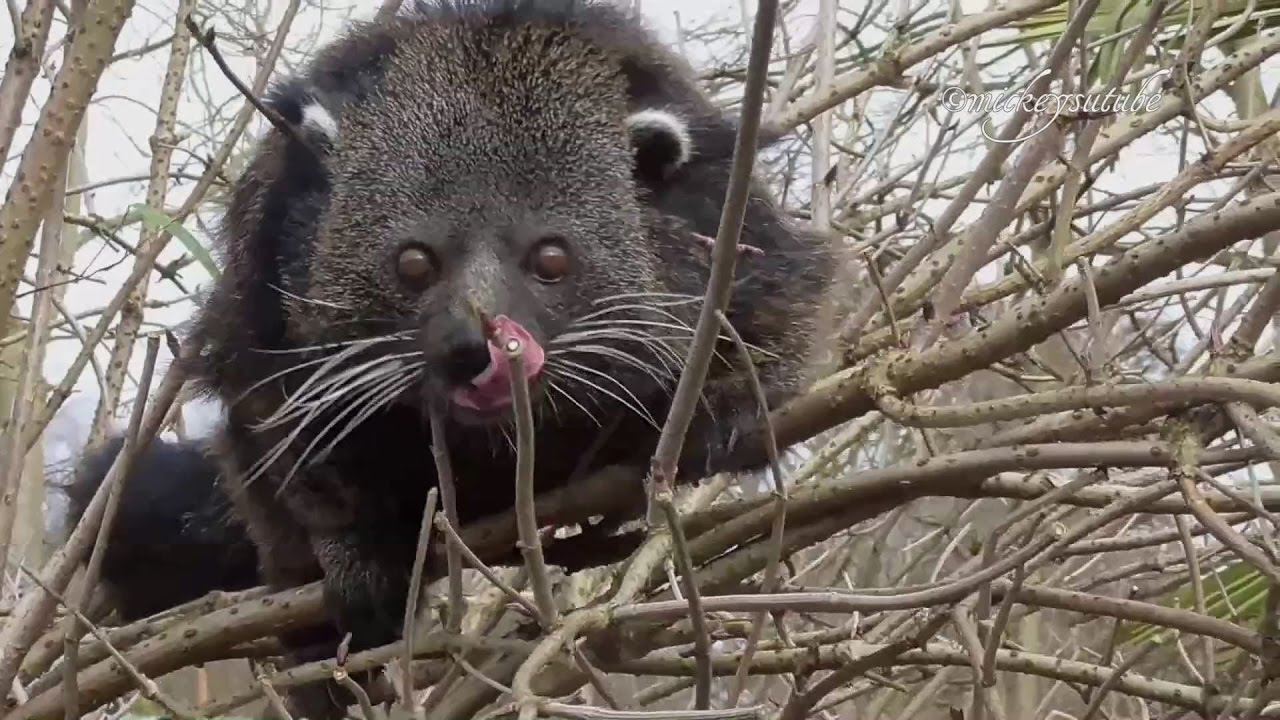This photograph depicts a small animal resembling a bear, perched among the branches of a leafless tree. The animal features dark fur, a round and sturdy body, and distinctive facial characteristics including long white whiskers, light coffee-colored round eyes, and small ears with white tufts. Its pink tongue is visible, giving the impression that it might be licking its chops. The photograph is a close-up shot, capturing the animal's detailed expression as it looks directly at the camera. The sky in the background is overcast, creating a white, muted backdrop. The tree's branches are brown and devoid of leaves, adding to the wintry atmosphere of the scene. In the top right corner of the image, there is some faint text, possibly the name of the photographer, though it is difficult to discern.